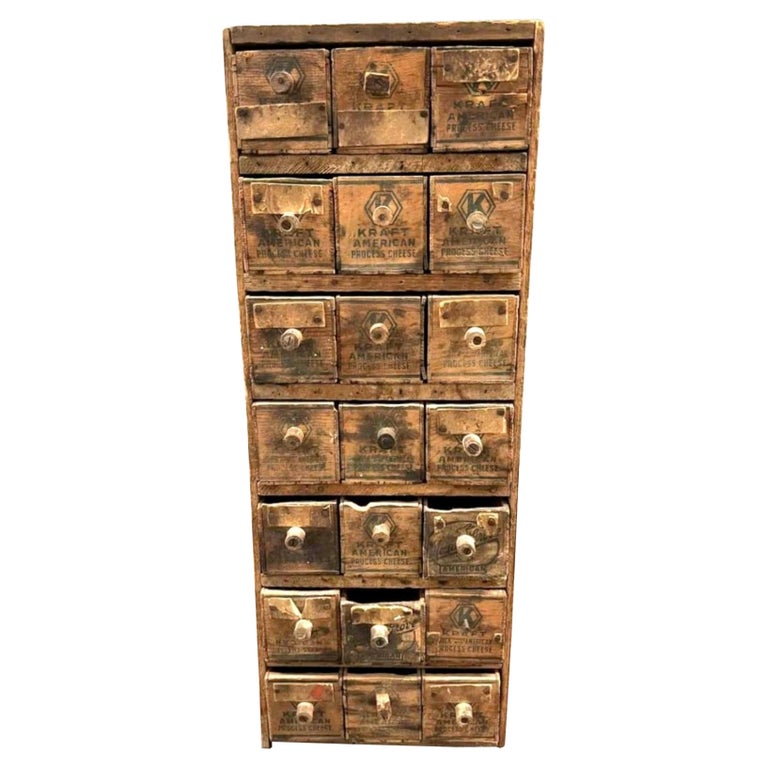The image depicts a vintage apothecary cabinet with a total of 21 small, narrow drawers arranged in seven rows of three. Each drawer has a white knob for pulling, though some knobs are uneven or mismatched, showing signs of wear and tear. The cabinet itself is an old, rusty brown with visible black spots in some areas, enhancing its aged appearance. Each drawer is labeled, but many labels are faded and difficult to decipher. Notably, one label on the second row, middle drawer, clearly displays the word "KRAFT." The cabinet's overall structure and worn-out state suggest it has seen extensive use over the years. The photograph is set against a white backdrop, highlighting the antique, somewhat dilapidated charm of the piece.